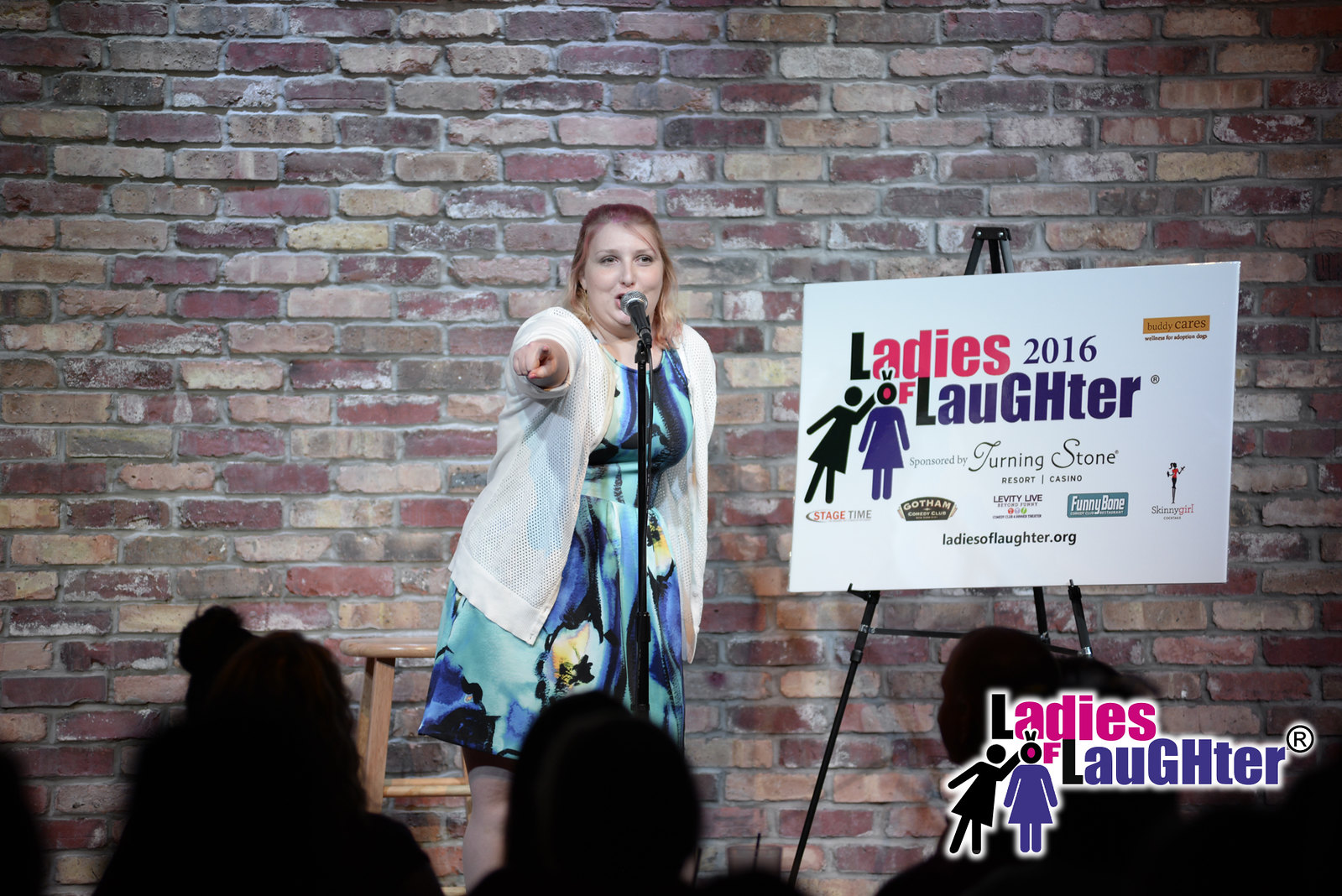The image portrays a woman performing stand-up comedy on a stage, framed by a rustic, multicolored red and yellow brick wall. She has red hair pulled away from her face and light skin, and she is adorned in a striking blue dress with abstract yellow flowers, complemented by a white wool jacket. The woman stands poised, pointing her left hand towards the audience while speaking into a black microphone. To her right, on an easel, is a white sign that reads "Ladies of Laughter 2016," with "Ladies" in pink and "Laughter" in purple. The sign also features a cartoon illustration of a woman hitting another outlined purple woman, and beneath it are various advertisements and sponsorships such as Turning Stone Resort Casino, Stage Time, Gotham Comedy Club, Levity Live Beyond Funny, Funny Bone, Skinny Girl Cocktails, ladiesoflaughter.org, and Buddy Cares Wellness for Adoption Dogs. At the bottom right of the image, the "Ladies of Laughter" logo is visible again. The audience is represented as dark silhouettes at the bottom of the image, their heads forming a front row as they attentively watch the performance.